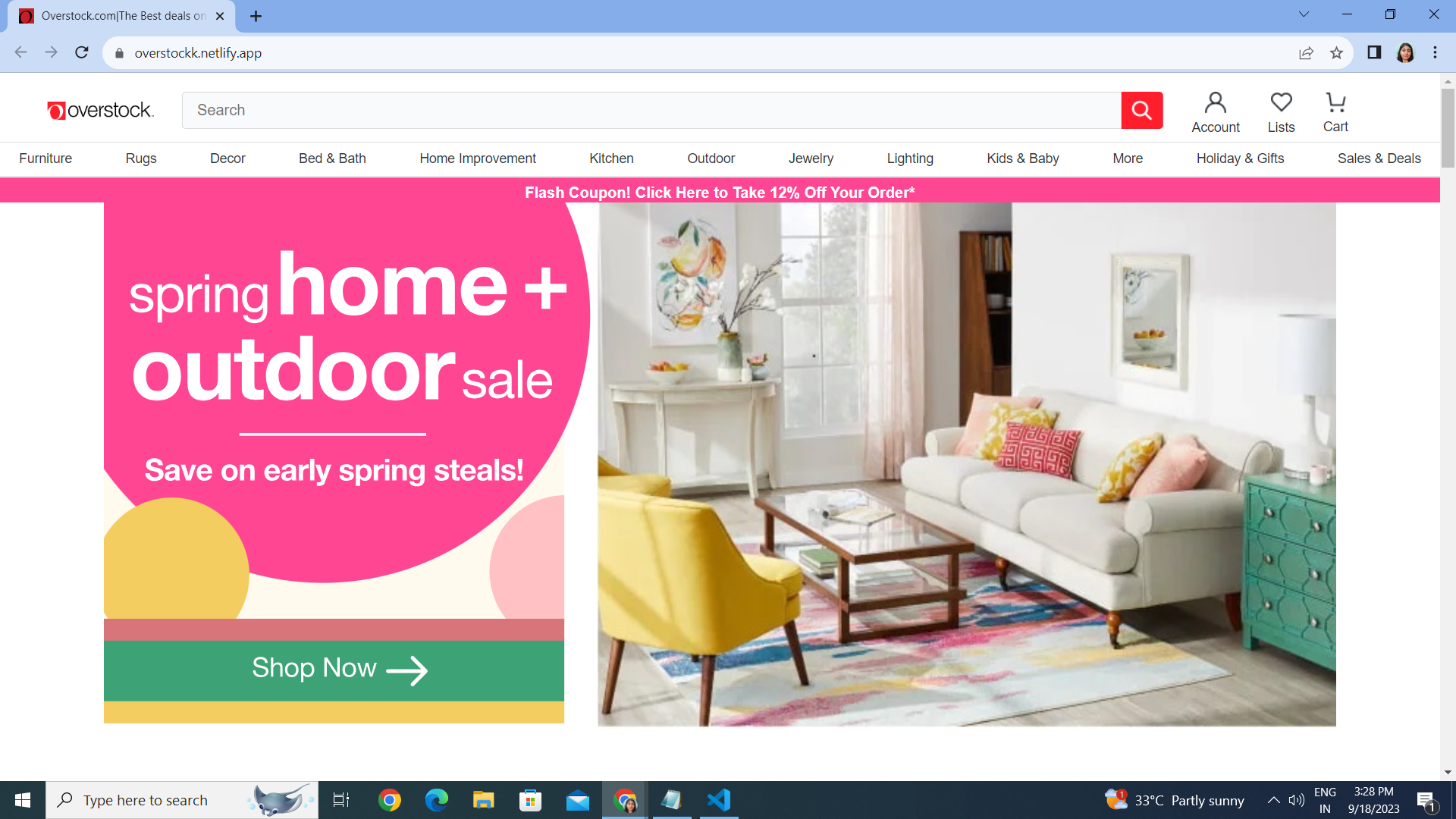This is a detailed screenshot taken from the company's webpage, Overstock.com, viewed on a desktop or laptop using the Chrome browser. The browser tab is labeled "Overstock.com: The Best Deals on the..." but the title is cut off. In the URL bar, the webpage address is displayed as overstock.netlify.app. On the right side of the browser toolbar, there is a profile image of a female face.

The Overstock website features prominently, with a lengthy search bar displaying a red border, followed by options for Account, Lists, and Cart. Beneath this, there is a horizontal navigation menu listing various categories including Furniture, Rugs, Decor, Bed & Bath, Home Improvement, Kitchen, Outdoor, Jewelry, Lighting, Kids & Baby, More, Holiday & Gifts, and Sales & Deals.

Central to the page is a promotional banner for the "Spring Home Plus Outdoor Sale" with a pink background and an Easter egg design theme, advertising discounts on early spring items. There is a "Shop Now" button in green and a "Flash Coupon" banner encouraging users to click for a 12% discount. The image within the banner depicts a cozy living room featuring two couches, suggesting the types of products on sale.